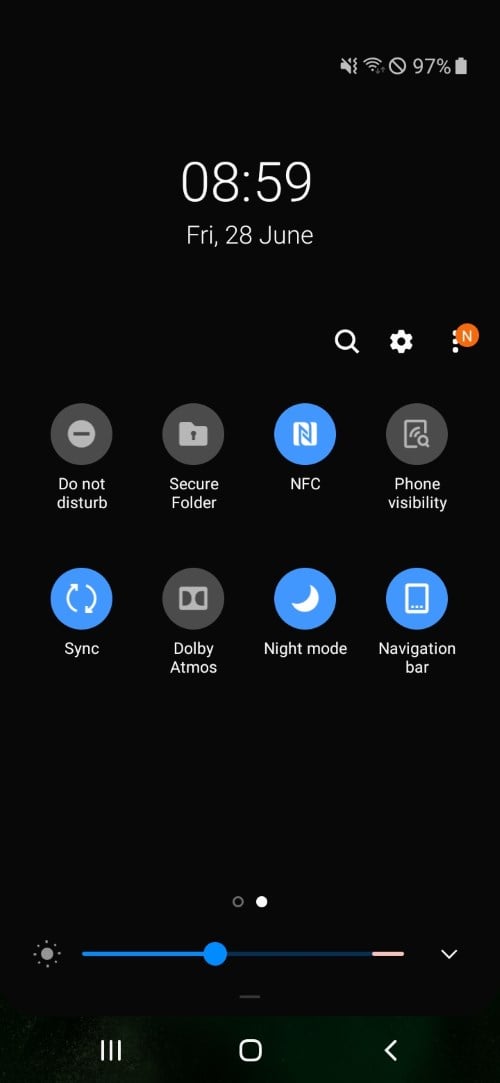This image depicts the home screen of a cell phone in a portrait orientation against a black background. 

At the top right corner, there are status indicators including a crossed-out audio symbol, indicating silent mode, followed by the internet signal icon. Next is a circle with a cross, resembling a no-entry sign, and a battery indicator showing 97% charge. Below these icons, it displays "08:59 Friday, 28 June," indicating the time and date.

Towards the upper-right section, there are three functional icons: a search button represented by a magnifying glass, a settings cogwheel, and the three dots symbol for additional options.

Beneath this row, there are four circular icons in a horizontal line. The first icon on the far left is labeled "Do not disturb." Next to it is an icon of a folder labeled "Secure Folder." Following this is an N logo representing "NFC" (Near Field Communication) and finally, an icon labeled "Phone visibility."

Further down, another row of four circular icons is present. These include "Sync," "Dolby Atmos," "Night mode," and "Navigation bar."

Below these icons sits a brightness adjustment bar, set to halfway. At the bottom of the screen, there are three navigation controls: three vertical lines, an icon resembling a television screen, and an arrow pointing to the left.